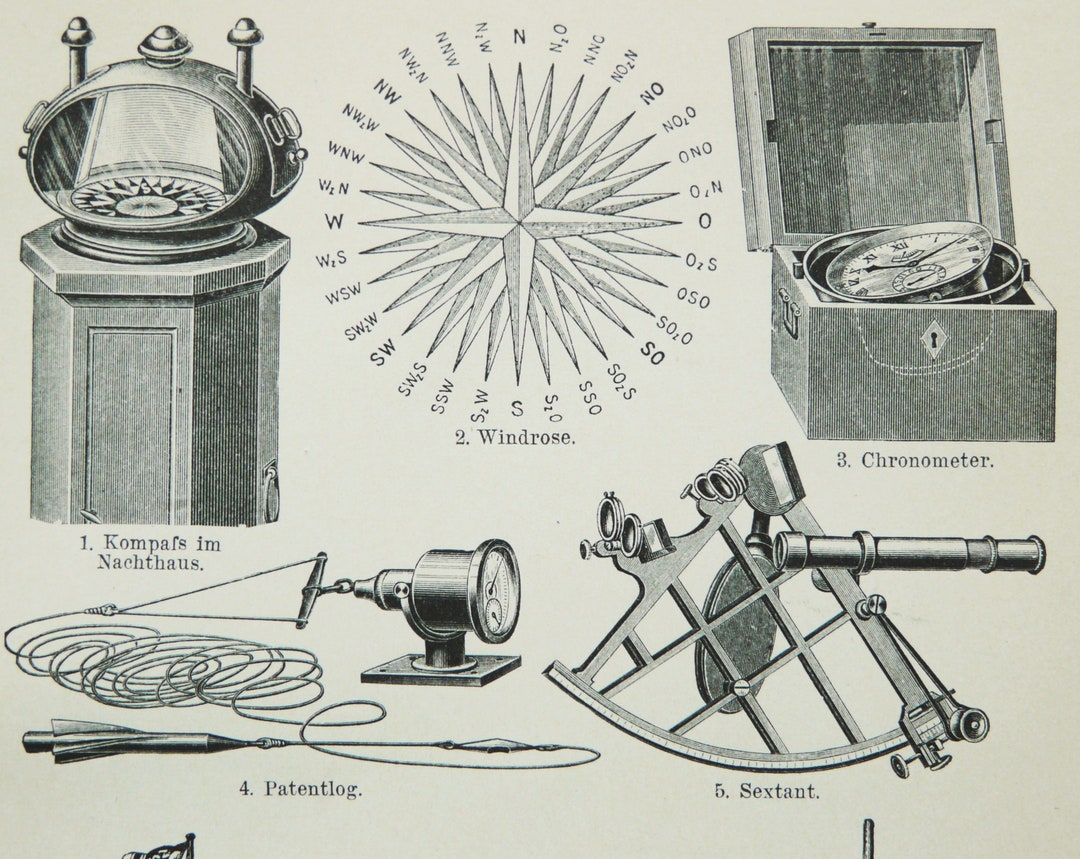This detailed antique drawing showcases a collection of vintage navigation tools, each intricately sketched with accompanying descriptions in German. In the upper left corner, there is a depiction of a traditional compass labeled "Kompass," nestled within what seems to be a protective casing. Adjacent to this, in the center, a diagram labeled "Windrose" displays compass headings, with detailed indicators marking cardinal directions. Moving to the upper right, the image features a "Chronometer," encased in a sturdy, lockable wooden box, highlighting its importance and vintage design. On the lower left side, labeled as number four, is a "Patent Log," resembling a rocket attached to a string, used historically for measuring a ship's speed. Completing the ensemble on the lower right is the iconic "Sextant," marked with the number five, a crucial tool for maritime navigation to determine angles and celestial locations. This drawing not only captures the historical essence of each instrument but also serves as a testament to the intricate craftsmanship and precision used in early navigation.